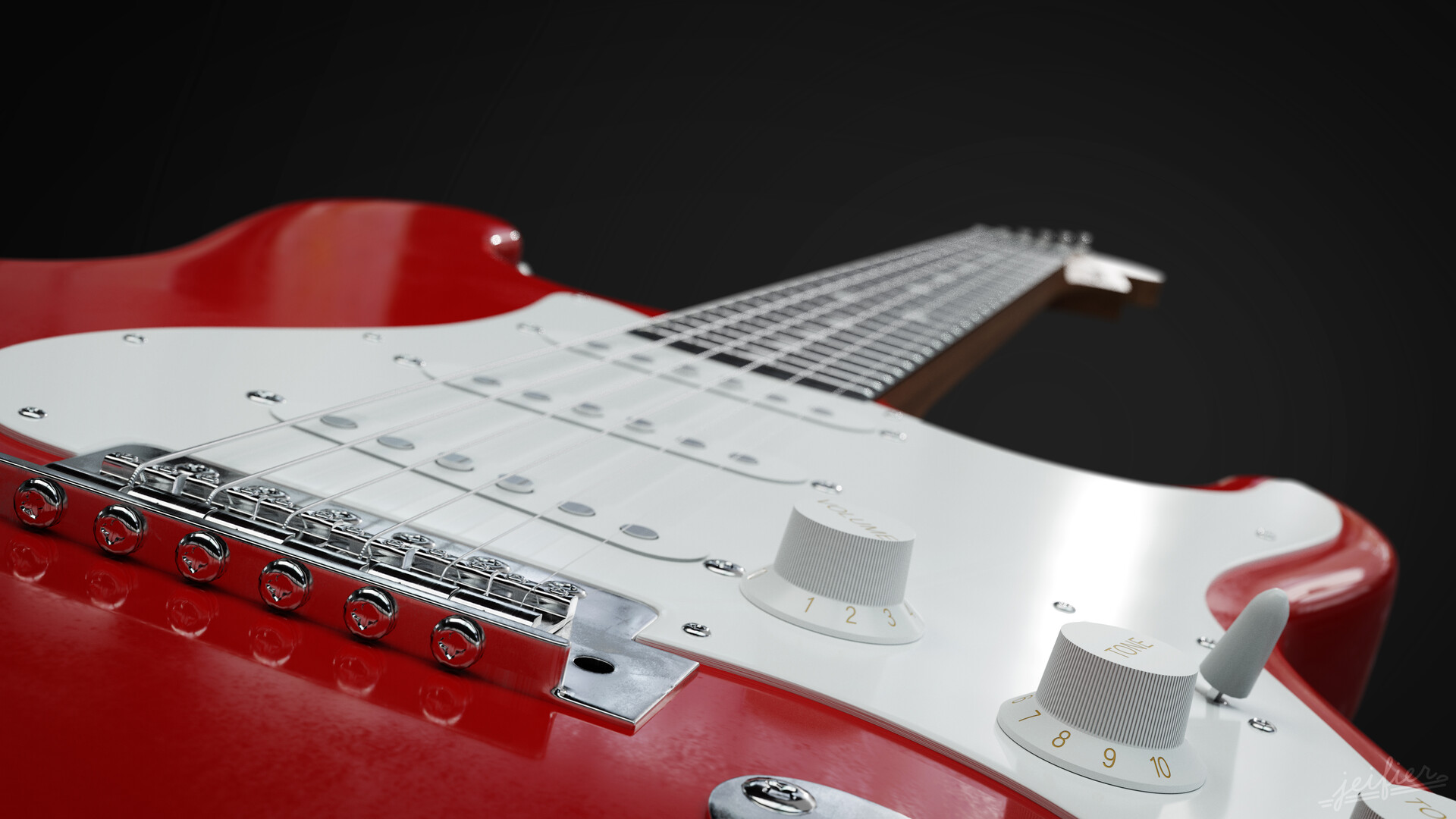The image captures a striking electric guitar set against a black background, with a close-up, tilted angle emphasizing its sleek and shiny design. The guitar's body features a vivid red color surrounding a white central section where the strings are. This white portion holds two control knobs and a distinctive whammy bar, all in white, which are used to adjust the guitar's sound. Chrome accents further add to its visual appeal. The lower part of the guitar starts in the bottom left corner of the frame and extends upwards, with parts of its red and white sections visible along both the lower left and right edges. The neck of the guitar extends into a black headstock adorned with a series of dots, adding almost a decorative touch to its functional design.